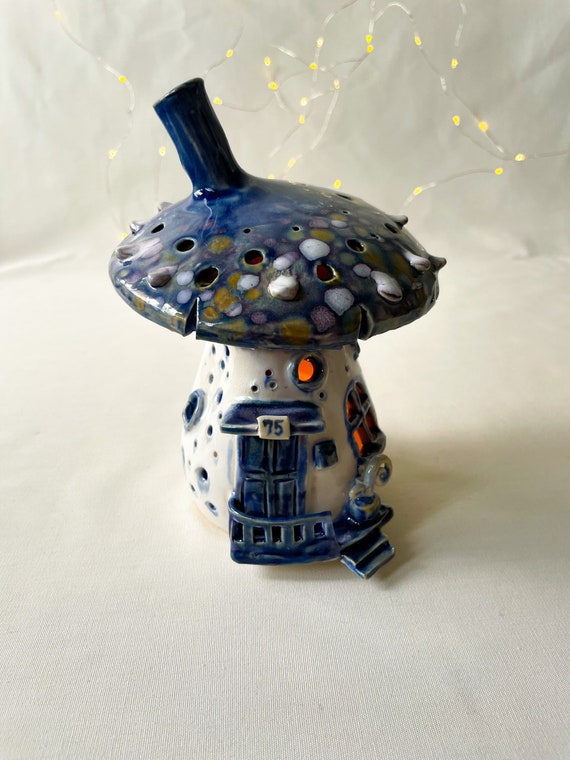The image depicts a detailed ceramic mushroom house. The house features a prominent blue mushroom cap with orange and white decorative spots, and a blue chimney protruding from the top left side. The body of the mushroom is predominantly white, complemented by several small carved-out windows that emit an orange glow, creating an illuminated effect. 

The front of the house boasts a blue-painted door marked with the number "75" on a white plaque. Above the door, there is a small blue balcony cover and a circular window. In front of the door, a blue railing adorns the entrance, accompanied by a set of steps on the right side. A tiny porch, featuring a squirrel and a plant pot, adds a whimsical touch. 

The background of the image includes some white cloth adorned with yellow fairy lights, enhancing the cozy and magical atmosphere of this miniature mushroom dwelling.